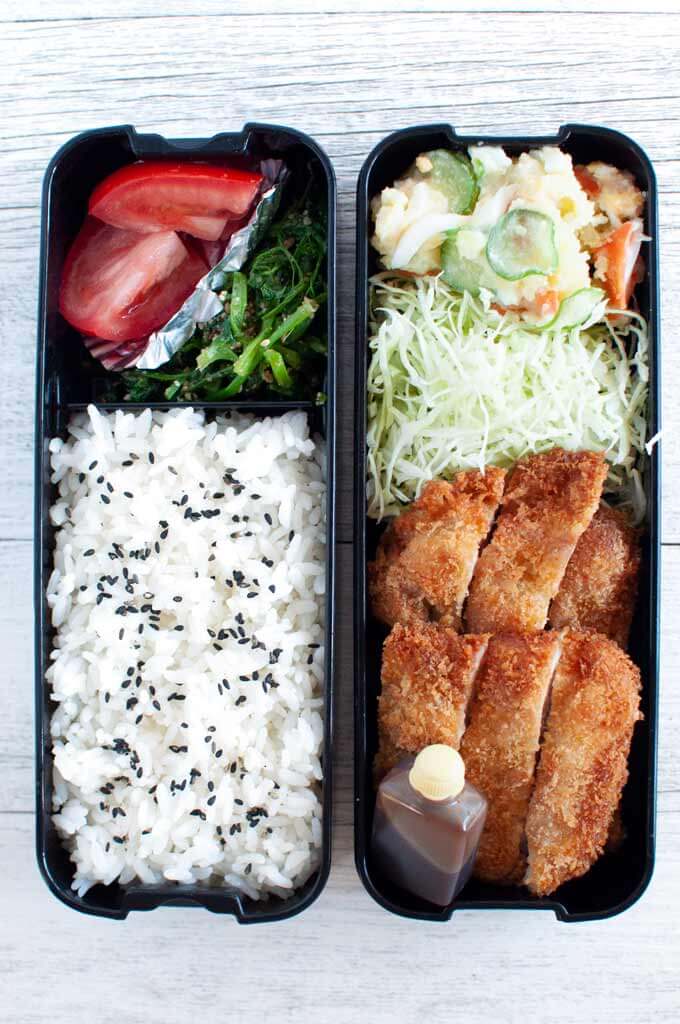Set against a bluish-gray wooden table, the image captures two rectangular black trays, arranged vertically in a top-down shot indicative of a food blogger's meticulous style. Each tray features a delightful variety of food items, beautifully organized within their compartments. 

On the tray to the right, fluffy white rice sprinkled with tiny black sesame seeds occupies the central partition. Adjacent to this, vibrant slices of tomatoes and another green leafy vegetable add a pop of color. The left tray showcases a crispy, golden-brown breaded piece of meat—either chicken or fish—accompanied by a small dish of savory sauce. Surrounding the protein, thinly sliced cabbage and a mixed salad featuring what appears to be celery, tomatoes, and possibly a white dressing complete the dish. The overall setting is bright, with excellent natural lighting highlighting the delicious array, making the viewer's mouth water.